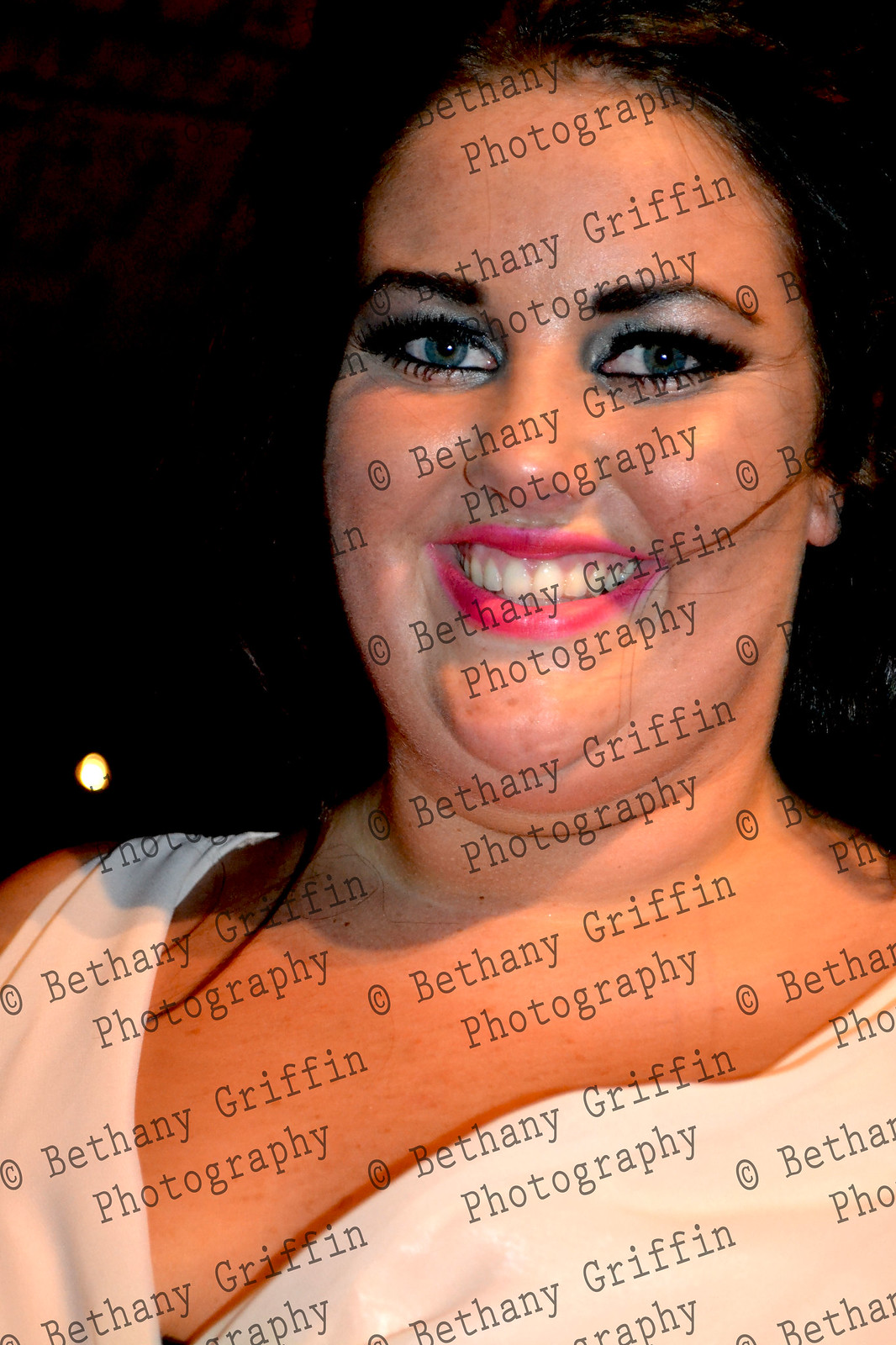The image is a portrait-style photograph of a smiling Caucasian woman with heavily applied makeup. Her eyebrows are thickly painted, her eyelashes clumped together with a substantial amount of mascara, and she has shiny gray eyeshadow and pinkish-red lipstick. She is wearing a white sleeveless shirt or dress, and her neck appears darker than her face. Only part of her ear, just the lobe, is visible. The background is completely black, possibly with a faint light, like a car headlight, barely discernible in the darkness. The photo is heavily watermarked with the text "Copyright Bethany Griffin Photography" repeated multiple times in a semi-transparent, dark font, which somewhat obscures the image.